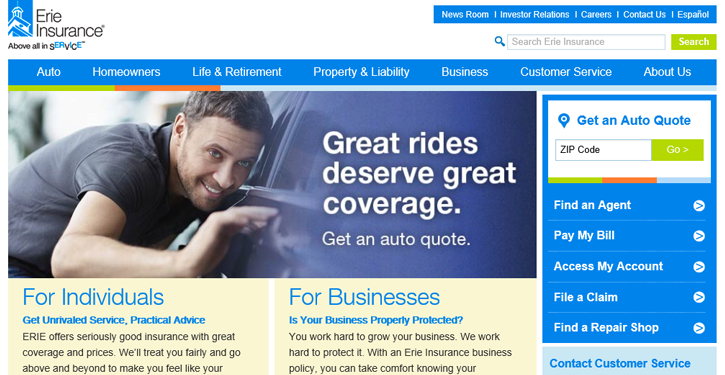The image showcases a website for Erie Insurance, with a clean, user-friendly interface. 

At the top is a prominent blue box featuring a small steeple icon and the text "Erie Insurance, Above All in Service." Adjacent to this box is a navigation bar in blue, offering quick access to sections such as Newsroom, Investor Relations, Careers, Contact Us, and Español. 

A search bar with a blue magnifying glass stands out next to a green "Search" button for easy access to site-wide information. Below the navigation bar, a menu lists various insurance options, including Auto, Homeowners, Life and Retirement, Property and Liability, Business, Customer Service, and About Us.

The main section of the page features a large image of a man in a gray shirt leaning against his car, gazing thoughtfully down its length. A prominent caption next to him reads: "Great Rides Deserve Great Coverage. Get an Auto Quote."

Further down, two sections cater to different audiences: "For Individuals" and "For Business." The individual section promises "Get Unrivaled Service, Practical Advice," and highlights Erie Insurance's commitment to offering excellent coverage and fair treatment, though the text cuts off mid-sentence. The business section questions if business properties are properly protected and emphasizes the hard work Erie puts into safeguarding businesses, encouraging users to get an insurance quote.

At the bottom, there are boxes for obtaining an insurance quote by entering a zip code, finding an agent, paying a bill, and accessing one's account, ensuring that all essential services are easily accessible.